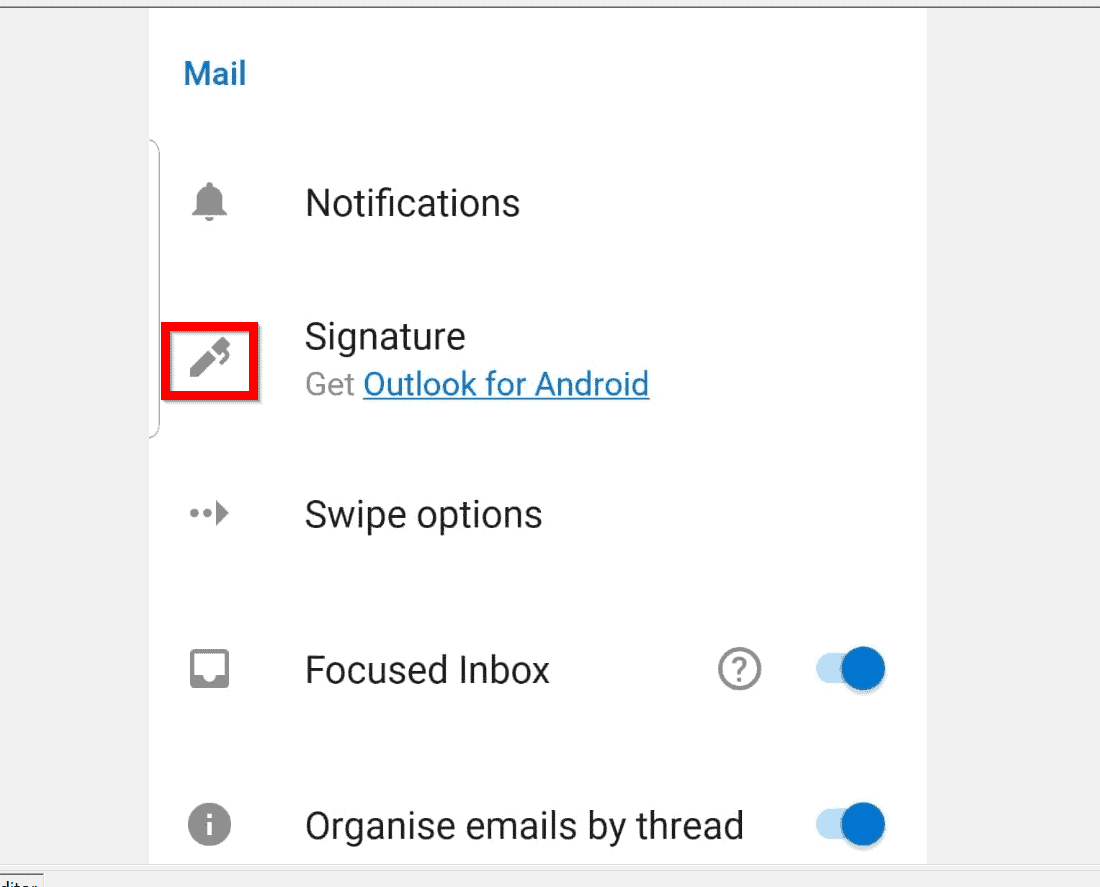The image is a detailed screenshot featuring a light gray background with a subtle border, framed from the upper left to the lower right, and the upper right to the lower left. In the upper left and bottom left corners, there are small icons indicating the display of additional elements, but the focal point of the image is a white card centralized within the frame.

The white card is designed to guide users through the process of managing their email settings, specifically focusing on the configuration of an email signature. Here's a detailed breakdown of the elements on the card:

1. **Upper Left Corner:** A blue mail icon.
2. **First Row:** A notifications bell icon accompanied by the word "Notifications".
3. **Next Row:** An edit pen icon enclosed in a red rectangle with the word "Signature" to its right. Below this is the prompt "Get Outlook for Android" in blue text.
4. **Following Row:** A right-pointing arrow denoting "Swipe Options".
5. **Subsequent Row:** The phrase "Focused Inbox" followed by a question mark inside a circle, indicating an option that is toggled on.
6. **Next Row:** An eye icon inside a circle with the text "Organize emails by thread," shown in an active status.

The highlighted "Signature" section, enclosed in a red rectangle, is intended to educate users on where to configure their email signature. Clicking on this area should allow the user to add a signature that will be automatically appended to all of their outgoing emails.

This descriptive guide provides a clear visual and textual reference for finding and setting up an email signature within the mail client, emphasizing its importance and ease of access.